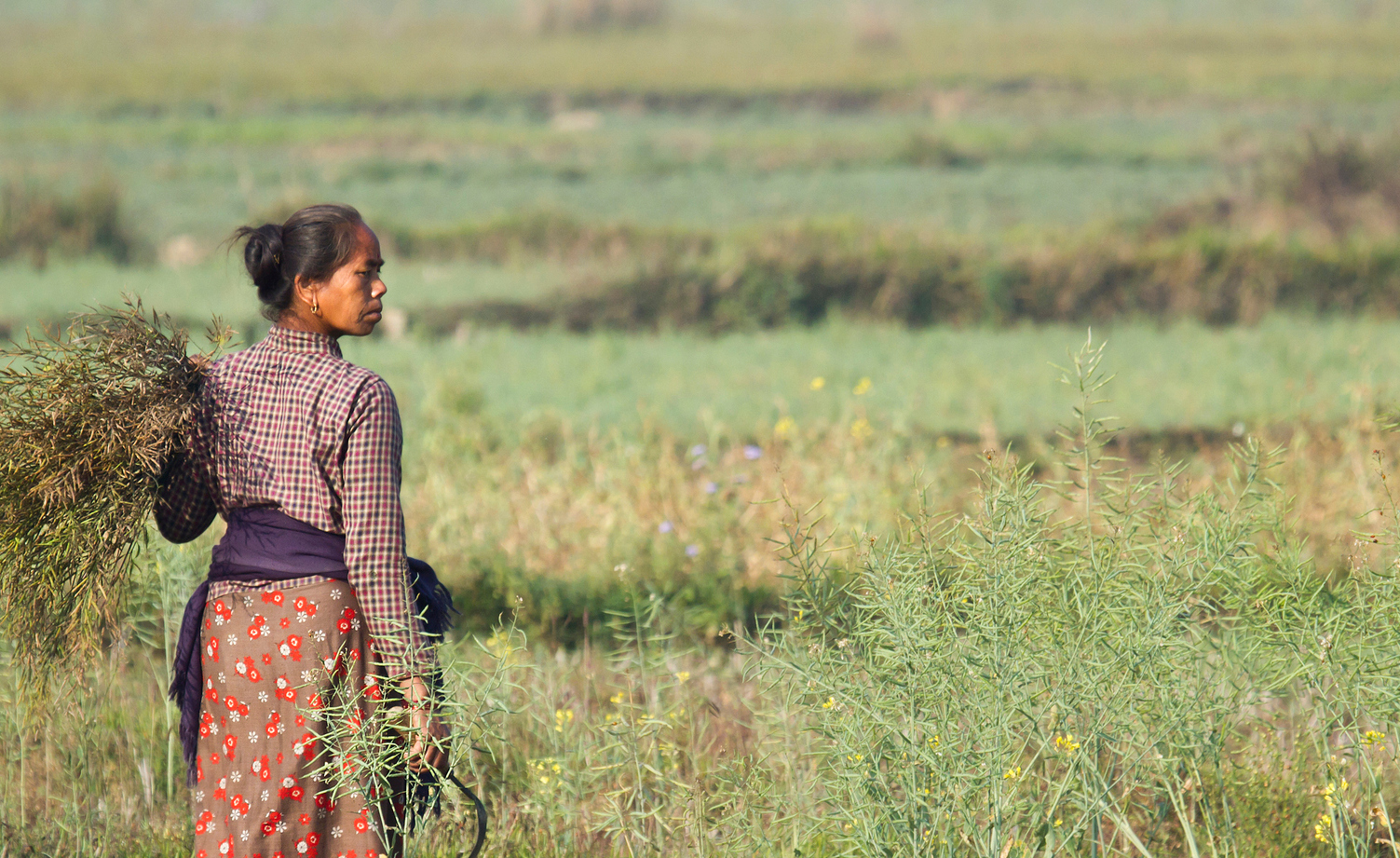In this image, we see a perhaps middle-aged woman of color, who appears to be Indian, standing in a picturesque, open field abundant with wildflowers and green plants, some adorned with small yellow blooms. Dressed in a checkered long-sleeved button-up shirt, a red and white skirt with a floral pattern, and a purple jacket tied around her waist (or blue-purple sash), she has her dark hair pulled up into a bun. Viewed mostly from behind, but with her head turned in profile, she holds a collection of native plants or branches in her left arm while grasping a sickle-like tool in her right hand. The scene's lower half is in crisp focus, showcasing the verdant and lively flora, while the upper half is more blurred, emphasizing the woman as the primary subject amidst the natural backdrop, suggesting she may be gathering these plants for artistic or decorative purposes.